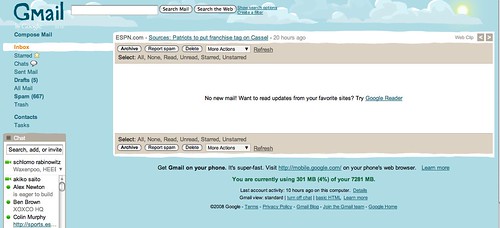The image showcases a Gmail inbox with a customized light blue background, featuring a sky theme with visible clouds at the top. The "Gmail" logo is prominently displayed on the left-hand side. Below it, various mail options are listed, including Inbox (highlighted in orange), Starred, Chats, Sent Mail, Drafts, All Mail, Spam, Trash, and Contacts. The interface shows no new mail in the inbox area, which has a white background, while gray options for archiving, reporting, deleting, or taking more actions are also visible.

An email from ESPN.com is visible, sent 20 hours ago, mentioning details related to franchises, although the content is somewhat blurred. Additionally, there is a chat bar on the left-hand side displaying online contacts, indicated by small green lights next to their names. At the bottom, information is available on how to get Gmail on mobile devices, including usage statistics in megabytes and links to Google's mobile website.